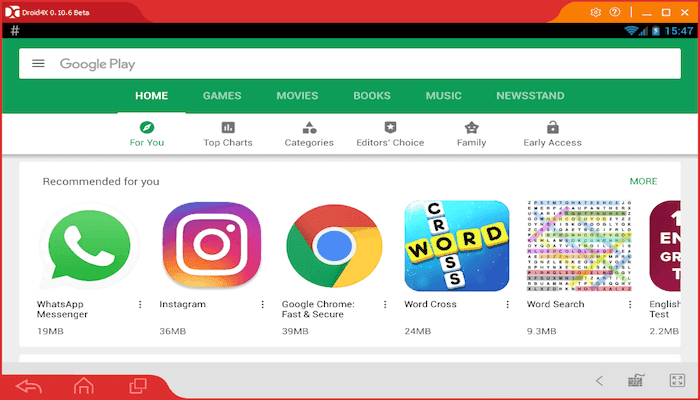The image displays a screenshot of the Google Play interface. At the very top, a prominent red bar is labeled "Droid DC Beta." Directly below, the Google Play search bar is visible. The primary navigation tabs include Home, Games, Movies, Books, Music, and Newsstand, with "Home" currently highlighted. Within the Home section, various subcategories such as 4U, Top Charts, Categories, Editor's Choice, Family, and Early Access are presented.

Highlighted apps in this section include WhatsApp Messenger, Instagram, Google Chrome (Fast and Secure), Word Cross, and Word Search. A portion of the text "English text" is also shown, though it appears incomplete. Each app's size is displayed: WhatsApp Messenger (19 MB), Instagram (36 MB), Google Chrome (39 MB), Word Cross (24 MB), Word Search (9.3 MB), and the English text app (2.2 MB).